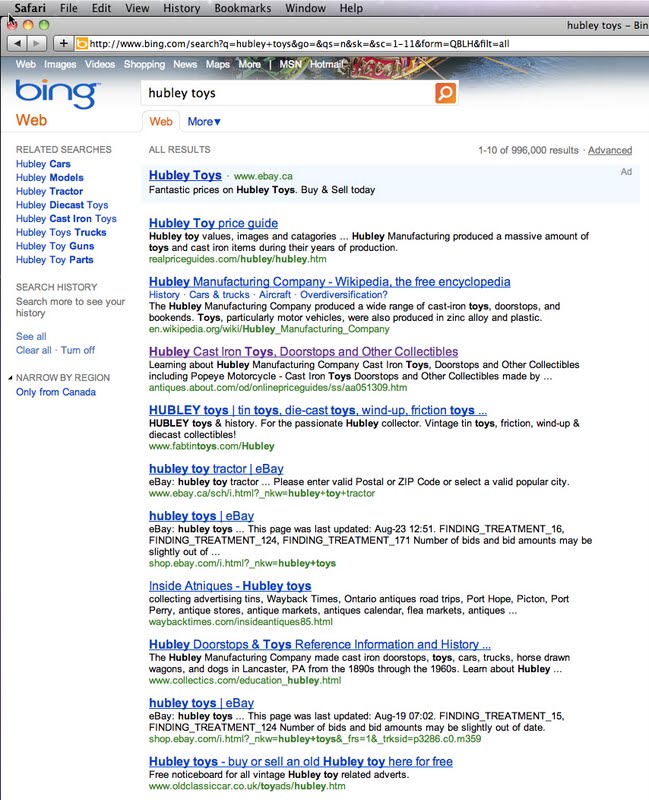This image captures the results of a Bing search for "Hubley toys." The search results include various websites related to Hubley, a renowned manufacturer of collectible toys. At the top, the listings include URLs such as www.ebay.ca, indicating online marketplaces where Hubley toys are sold. The search results also highlight a Hubley toy price guide and a Wikipedia entry for the Hubley Manufacturing Company. The Wikipedia snippet describes the company as a producer of a wide assortment of cast iron toys, doorstops, and bookends, as well as motor vehicles made from zinc alloy and plastic. Further down the search results, there are mentions of Hubley's cast iron toys, doorstops, and other collectibles, along with categories like tin toys, die-cast toys, and wind-up friction toys. Additional links point to Hubley toy tractors and more eBay listings for Hubley toys. An orange search bar is positioned in the middle top area of the page, ready for any new queries.